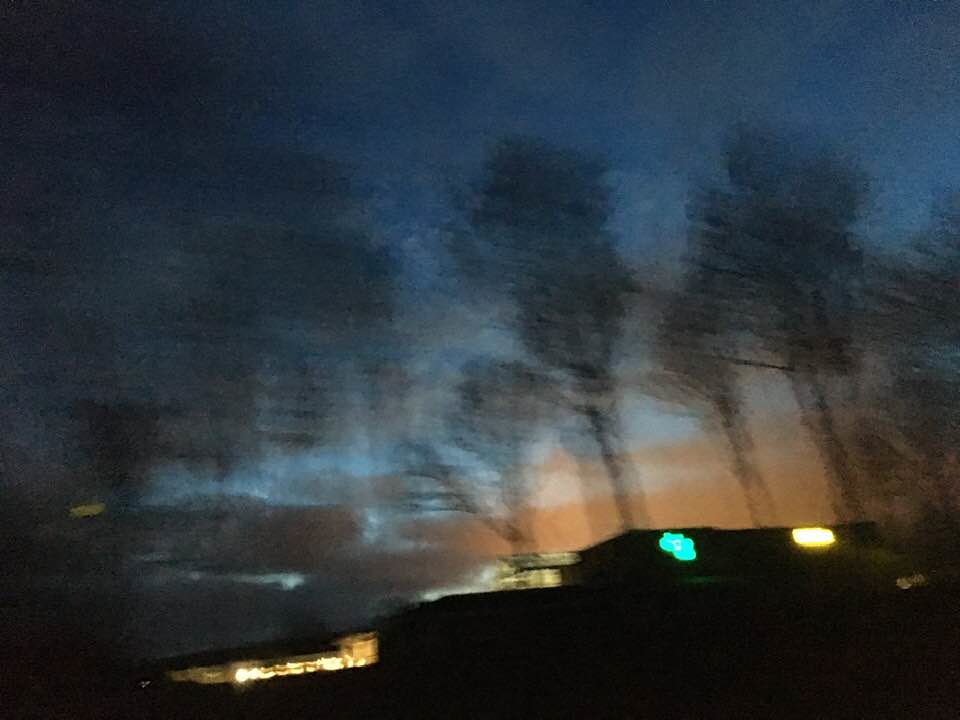A blurred color photograph likely taken from inside a moving car, capturing the serene beauty of a sunset. In the foreground, a dark hill spans the bottom of the image, dotted with streaks of yellow and blue lights that suggest distant houses or buildings. The sky, which begins on the left side with ominous, dark clouds, transitions into a stunning array of colors. To the right, vibrant streaks of orange give way to hues of light blue, eventually blending into deeper blue tones at the top of the frame. Barely discernible black lines hint at trees, devoid of detail, adding an artistic touch to this tranquil, picturesque scene.